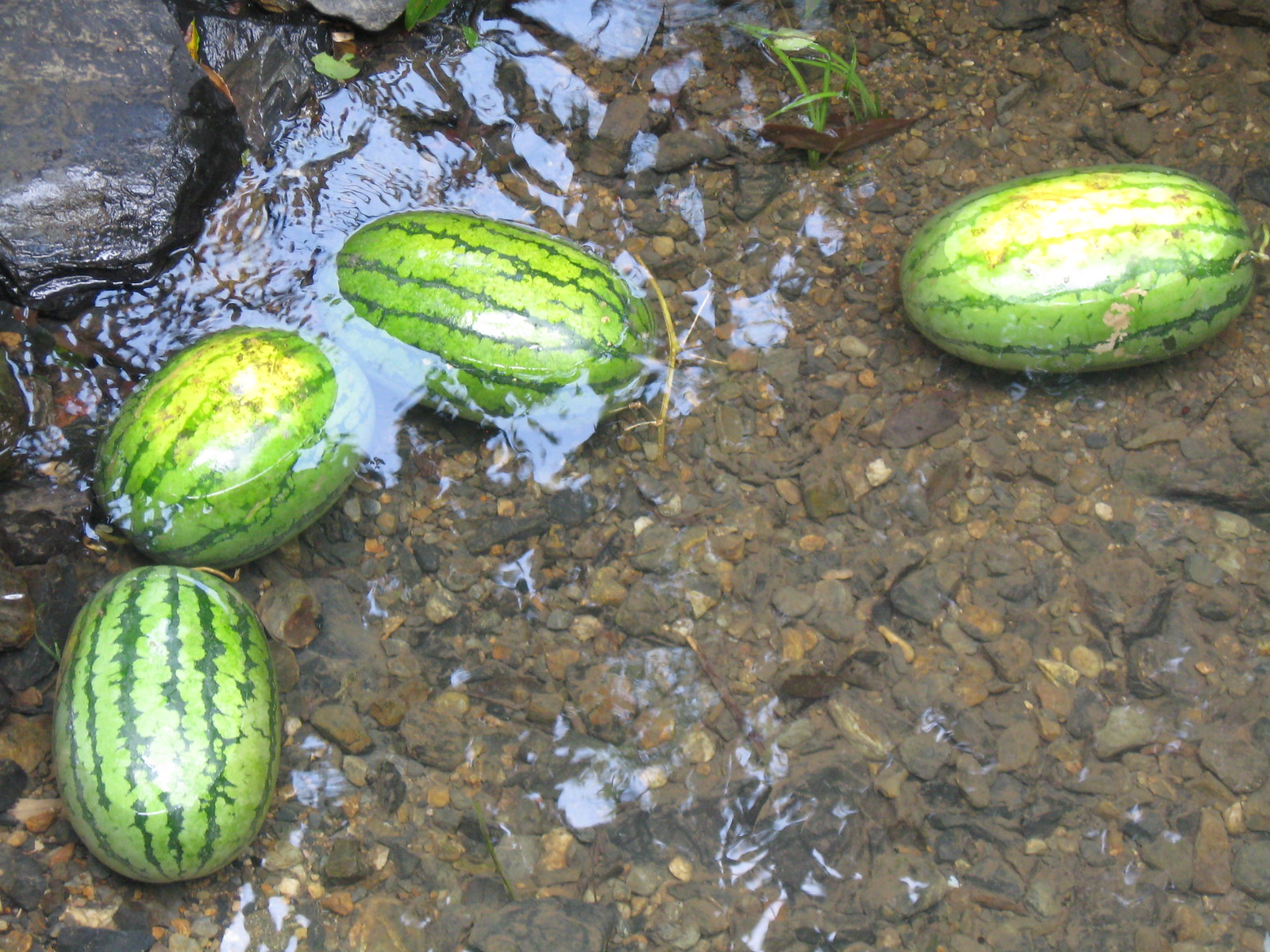In this detailed photograph, a picturesque creek bends through a serene landscape, its clear waters revealing a bed of variously colored pebbles—brown, tan, and white—interspersed with grassy patches and bits of leaves. In the clear stream, four large, green watermelons with dark green stripes, and two featuring yellow circle spots, float, with their tops just above the surface, suggesting buoyancy. Three of the watermelons are grouped closely on the left side, while the fourth is positioned towards the top right. A stick lies beside one of the watermelons, adding to the natural elements of the scene. The top left corner of the photograph shows a bank with larger rocks, some of which remain dry due to the lower water level. A strong sunlight reflection makes it harder to see beneath the water in that area, adding a shimmering effect to the idyllic creek setting.